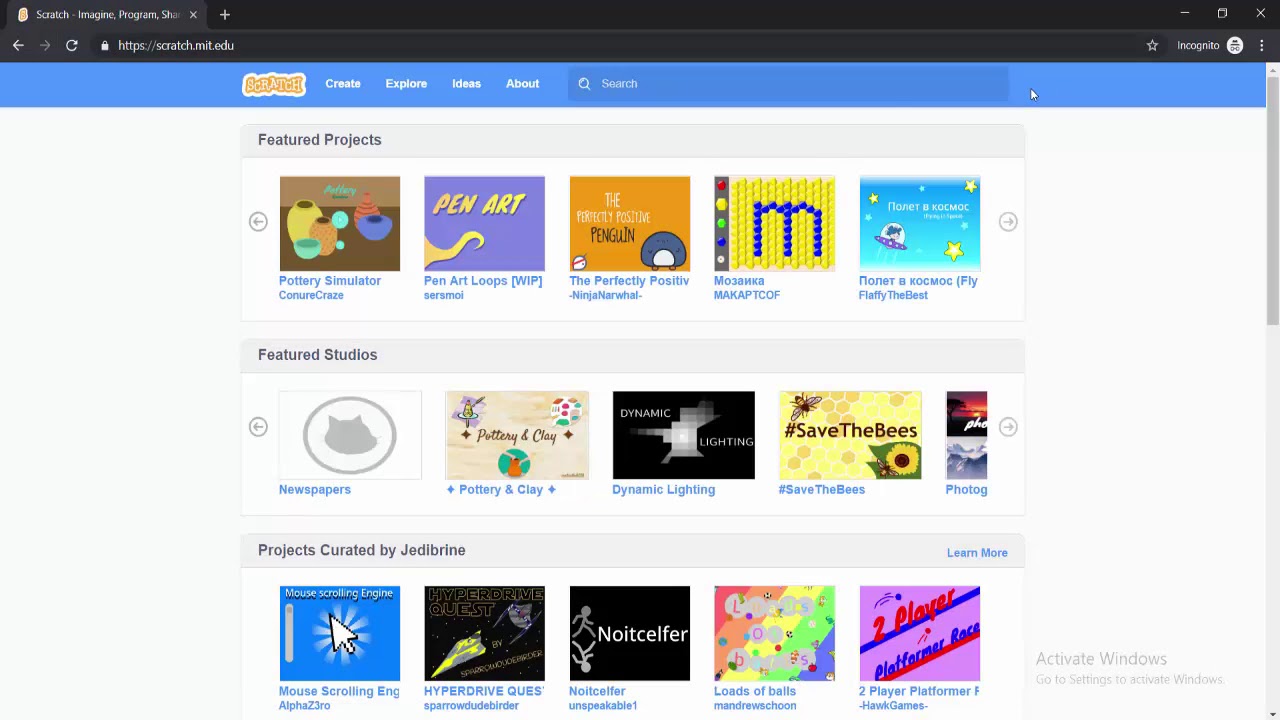This screenshot captures a web browser interface with distinct visual elements. The browser features a dark gray header that frames the content below. The primary web page underneath showcases a blue header design. On the left of this header, bold, white text with an orange outline, further encased in another white outline, prominently displays the word "SCRATCH" in all caps. Adjacent to this, to the right, are navigation links labeled "CREATE," "EXPLORE," "IDEAS," and "ABOUT." Continuing rightwards is a slightly darker blue search box with rounded corners. This search box features a white magnifying glass icon on the left and the word "SEARCH" in white text on its right side. Nearby, outside the boundaries of the search box, is a white triangular cursor outlined in black.

Directly below, the body of the web page presents a light gray background. In the bottom right corner, dark gray text states "ACTIVATE WINDOWS," with smaller text below advising, "GO TO SETTINGS TO ACTIVATE WINDOWS." The top center of this page includes a slightly darker gray rectangular header, which extends into a white rectangular pane beneath it. This header contains dark gray text on the left reading "FEATURED PROJECTS," with adjacent blue text on the right instructing "LEARN MORE." Below this header are two additional panes of the same width, labeled "FEATURED STUDIOS" and "PROJECTS CURATED BY JEDIBRINE." Each of the first two panes is equipped with light gray arrows on either side, pointing left and right, respectively, indicating a carousel feature.